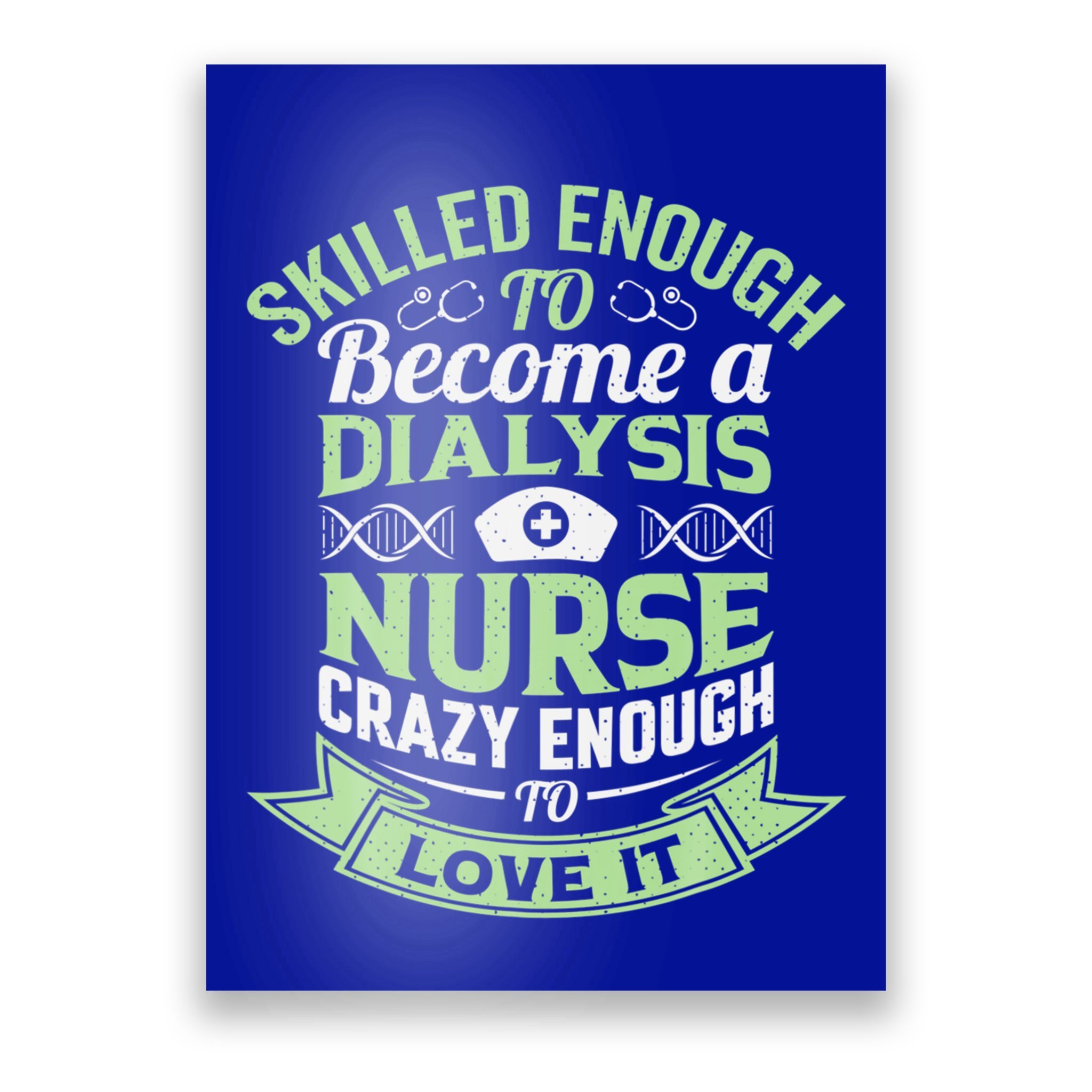This digital design, suitable for a t-shirt or sign, features a dark blue background with an arrangement of green and white text conveying a motivational message. At the top, in a curved, plain font of light green, the phrase "SKILLED ENOUGH" is displayed. Beneath it, a smaller, more cursive font spells out "TO" in white, flanked on either side by small stethoscope graphics. Following that, "BECOME A" is printed in a white, cursive font. 

The word "DIALYSIS" is prominently shown below in light green text, and directly underneath it, a pair of DNA hexagon icons frame a small white nurse’s hat with a cross. The sequence concludes with "NURSE" in light green, followed by "CRAZY ENOUGH" in white. Another white cursive "TO" precedes a light green banner at the very bottom, within which the words "LOVE IT" are centered in blue print. The overall layout forms a cohesive and encouraging message: "Skilled enough to become a dialysis nurse. Crazy enough to love it."